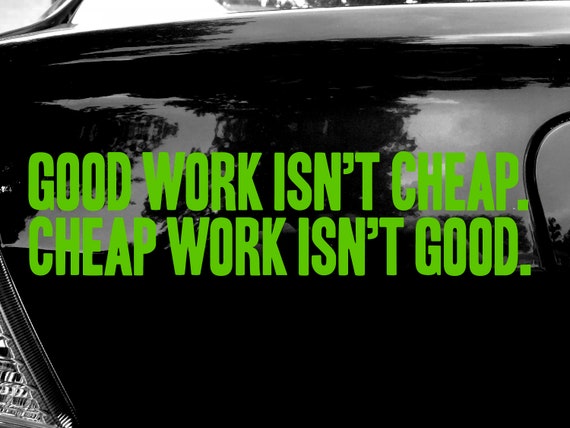The image is an extreme close-up of a glossy, black surface, likely the back of a car, reflecting light and showing the mirrored images of trees and bushes. The surface features bright green text centered horizontally, stating, "Good work isn't cheap. Cheap work isn't good." To the lower left side of the image, a small metal grill can be seen. On the right side, there's a semi-circular indentation, possibly the gas tank door. This reflection-heavy scene includes subtle details such as faint clouds, further adding to the depth and texture of the surface.